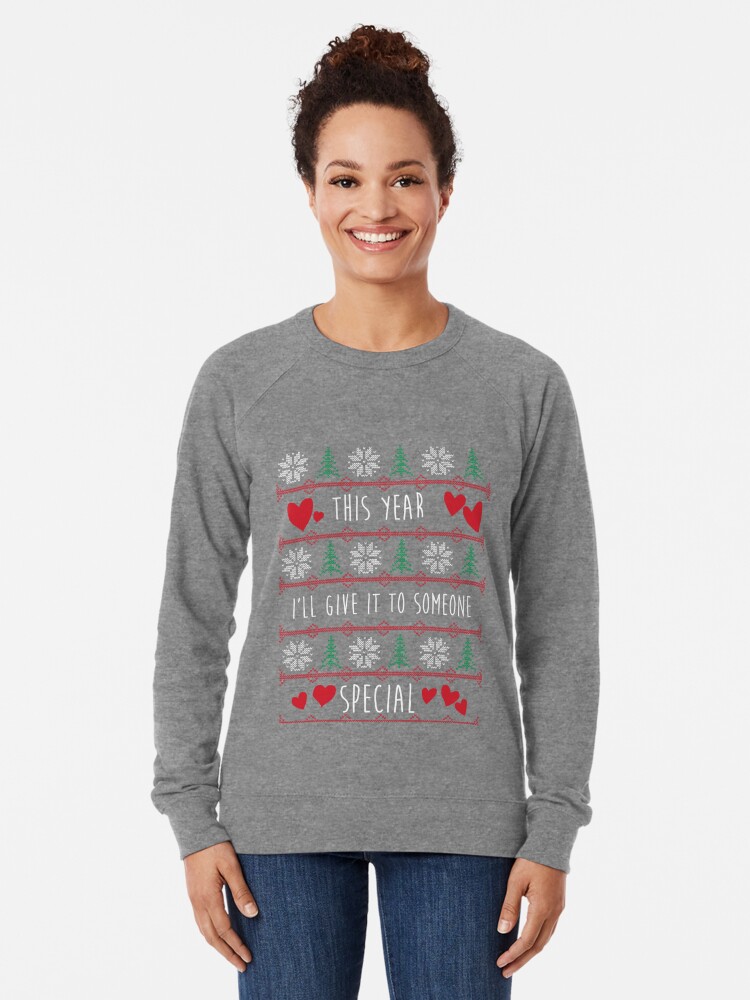In the picture, a woman with dark hair, styled in an updo, stands against a white wall. She is dressed in blue jeans and a long-sleeved heather-gray sweatshirt. The sweatshirt features a festive Christmas design with poinsettias and green Christmas trees interspersed with snowflakes. It reads, "This year I'll give it to someone special," with hearts surrounding the phrases "this year" and "special." The woman, who appears to be of mixed-race heritage with light-colored skin, exhibits a cheerful smile and looks directly at the camera. Her hands rest comfortably by her sides, enhancing the relaxed and joyful atmosphere of the image.